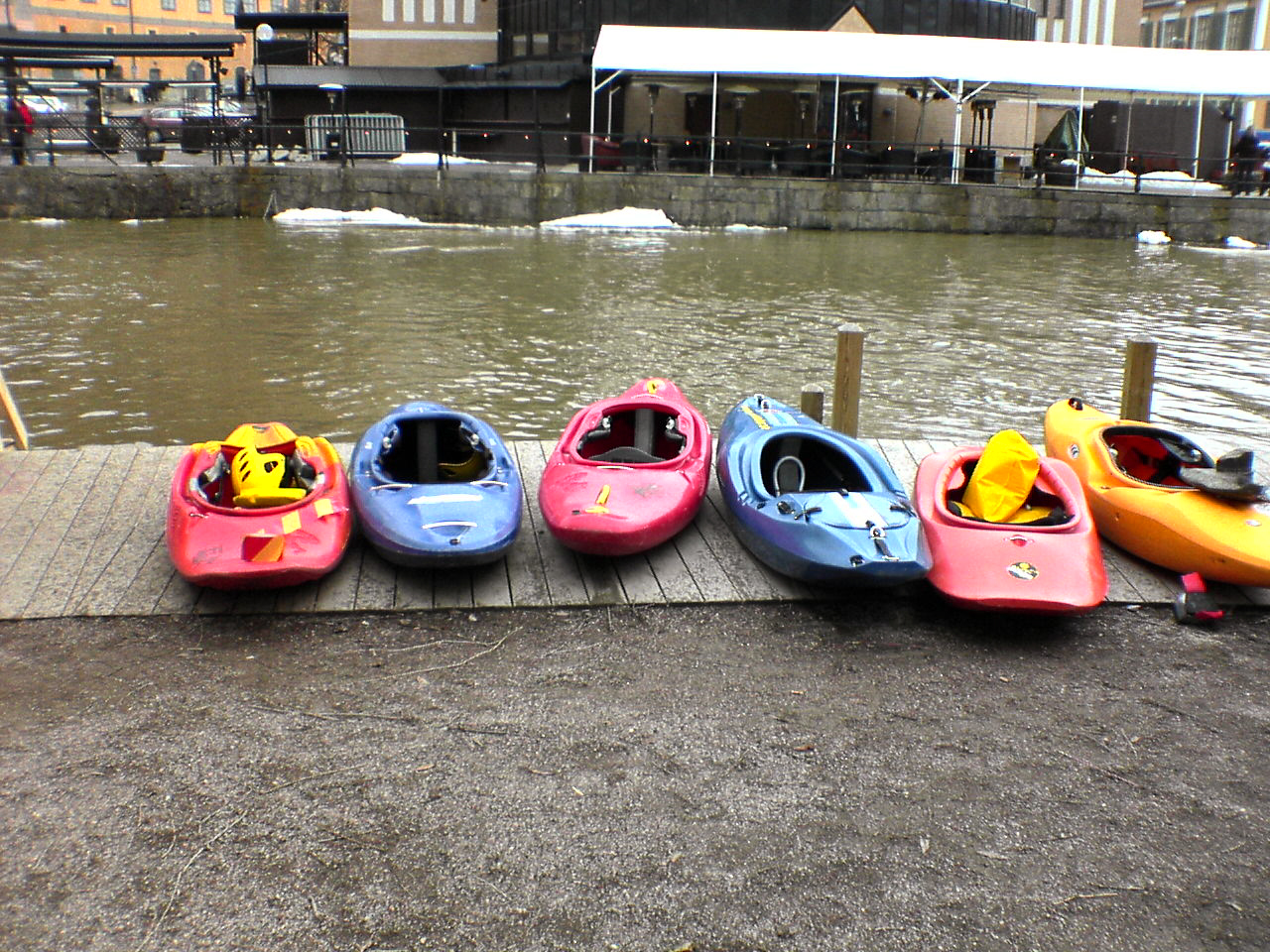In this vibrant, color photograph taken in a portrait orientation, we see an idyllic outdoor scene centered around a wooden pier that extends from a paved walkway in the forefront. The walkway joins a stretch of gravel or sand, forming the base of the scene. Atop the pier, there are six small plastic kayaks arranged as if prepared for a competition: three pink, two blue, and one yellow. Notably, one of the red kayaks contains a yellow bag, and another has yellow equipment. Rising from the water beside the pier, posts are visible, commonly used to moor boats. Beyond the kayaks, stretches a mucky greenish lake that leads to the distant shoreline, which is lined by a brick seawall. Across the water, several tall buildings are partially obscured by a large white canopy structure, which is part of a covered outdoor facility equipped with chairs. The entire scene is bathed in natural light, capturing the serenity and subtle activities of this inviting waterfront area.